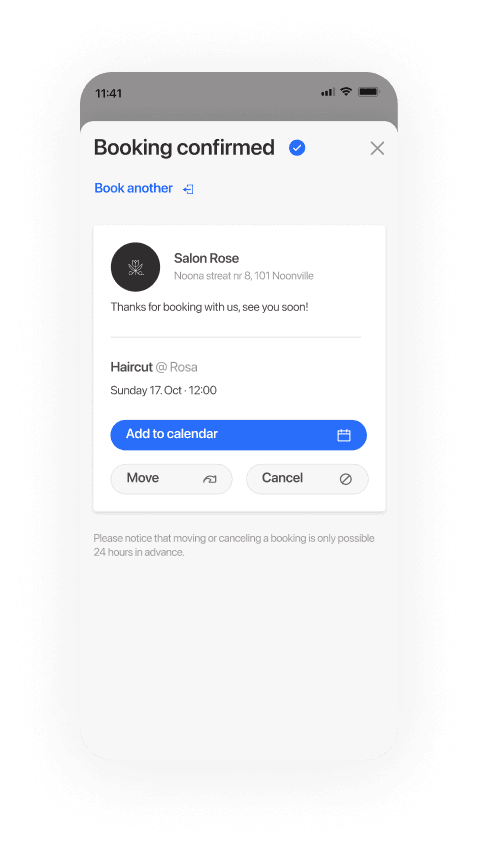The screenshot displays a well-organized booking confirmation page on a cell phone screen, captured at 11:41, with no indication of AM or PM. The phone features a fully charged battery, active Wi-Fi signal, and cell phone connectivity, all displayed prominently in the upper right corner. 

Below these indicators, the text "Booking confirmed" appears in bold black letters, accompanied by a blue circle with a white check mark and a gray 'X' icon on the right side. Beneath this confirmation text, a blue hyperlink labeled "Book another" invites further reservations. 

Next, a black circle appears, detailed with the text "Salon Rose, Nuna Street, 8101, Noonville," identifying the booked venue. Following this, the message "Thanks for booking with us. See you soon." conveys appreciation and anticipation for the upcoming appointment. 

Further down, specifics of the appointment are laid out: "Haircut at Rosa on Sunday, 17th of October at 12 o'clock." An option to add this appointment to the calendar is presented through a blue button with white text reading "Add to calendar." 

At the bottom of the screen, two additional action buttons are visible: a "Move" button and a "Cancel" button. The screen concludes with a disclaimer: "Please notice that moving or canceling a booking is only possible 24 hours in advance." 

This detailed view encapsulates all essential information regarding the appointment, offering convenient options for managing the booking.